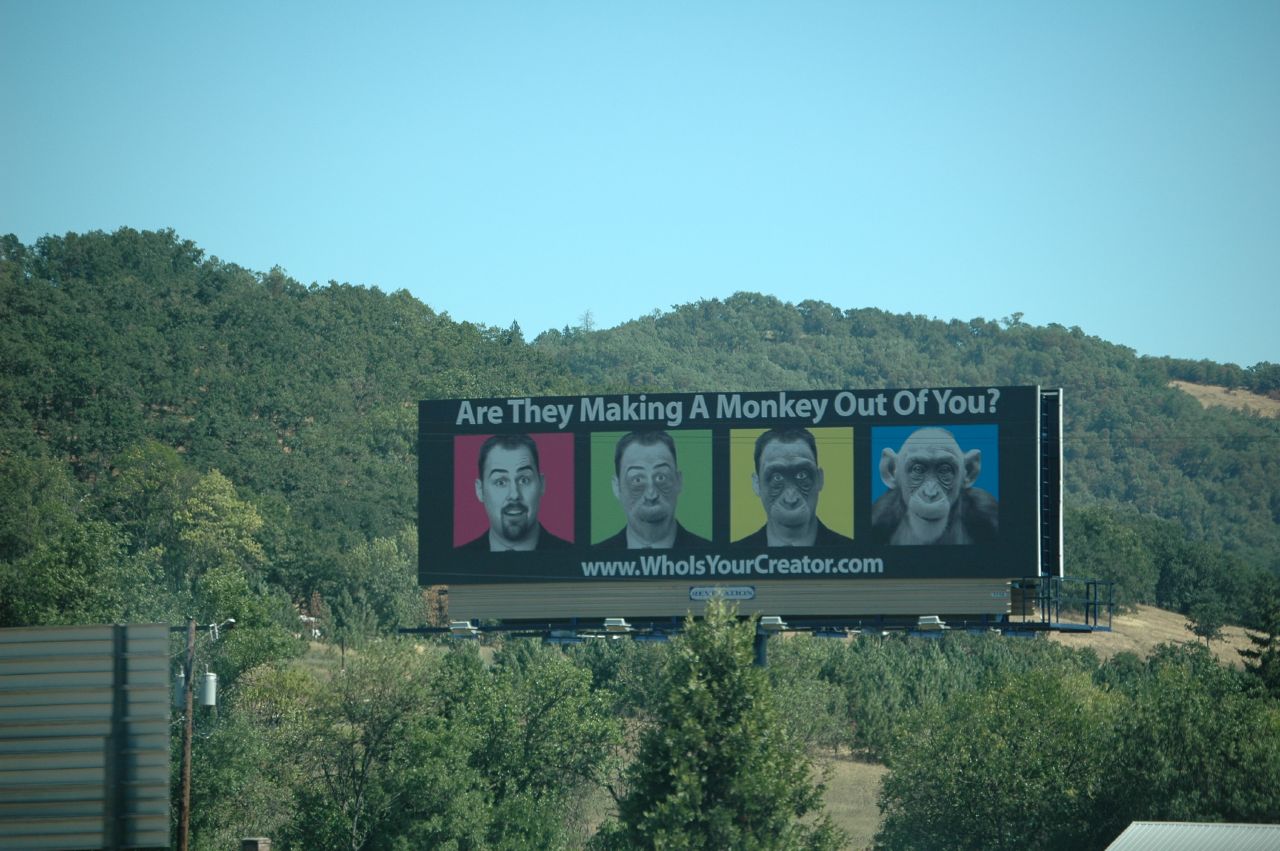The billboard depicted in the image features a provocative sequence of four images designed to catch the eye and provoke thought. The leftmost panel displays a man against a red background. As the viewer's gaze moves to the right, the next panel shows the same man beginning to exhibit monkey-like features, set against a green background. The transformation continues in the third image, where the man's features are even more simian and the background is yellow. The final image on the far right is a fully realized chimpanzee against a blue background.

The tagline above the sequence reads, "Are they making a monkey out of you?" Beneath the images, a website URL is displayed: www.whoisyourcreator.com. 

Adding to the billboard's intriguing and somewhat isolated presentation is its setting—it stands alone amid sparse wilderness, surrounded by trees, patches of grass, and areas of exposed dirt. This suggests a remote location, likely alongside a highway cutting through the countryside. The contrasting natural environment enhances the striking visual and thematic impact of the advertisement.